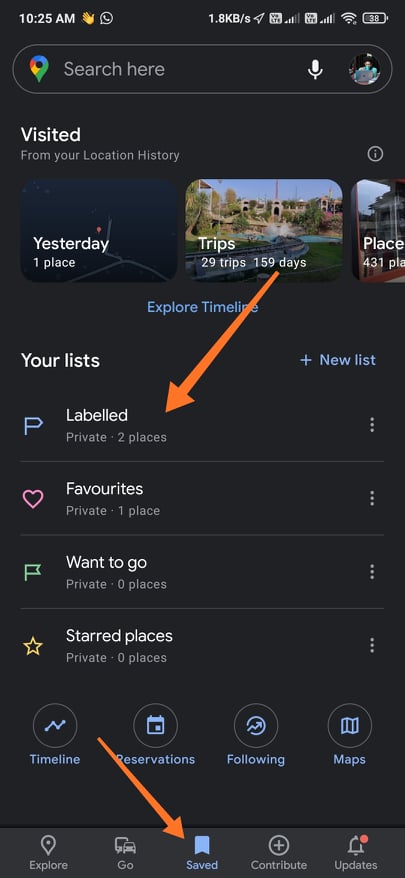A screenshot from a user's smartphone interface, showcasing various app elements and icons. The timestamp reads 25 AM, accompanied by an icon that resembles a clapping or waving hand and the WhatsApp logo. To the right of these icons, it displays "1.8 KB/s" and a send icon. The top-right corner displays indicators for LTE, half signal strength, Wi-Fi signal, and battery power at 38%.

At the center, the Google logo is visible above a search box containing a microphone icon and the user's image. Below this, white text reads "Visited" and beneath it, "From your local history." It provides details such as "Yesterday, one place," "29 trips," "159 days," and "431 places." Next to "Trips" is an image representing a vacation resort, while "Yesterday, one place" features a map icon.

In blue text below these details, it says "Explore Timeline," with "Your Lists" written in white to the right. Further down, there is a vertical list labeled "Private," encompassing "Two places," with three gray dots to the right. Other list categories include "Favorites," "Want to go," and "Starred places," all marked private with corresponding zero places, each accompanied by three gray dots.

Near the bottom, multiple buttons are listed: "Timeline," "Reservations," "Following," "Maps," and at the bottom navigation bar, an orange arrow highlights the "Saved" section. Moving left, icons for "Explore," "Go," "Contribute," and "Updates" are displayed, with a red dot indicating new updates available.